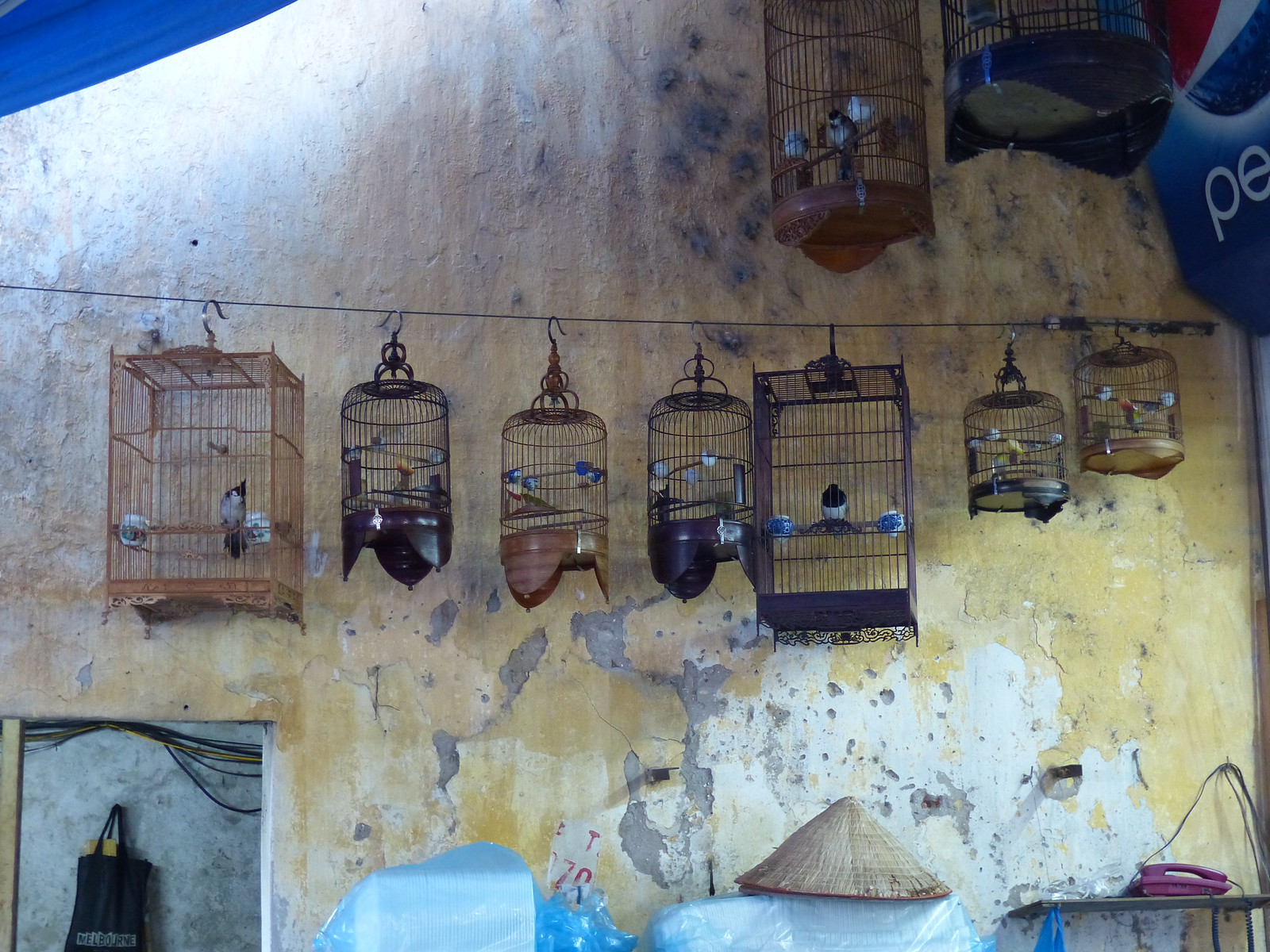This vibrant photograph captures the weathered exterior of an old building, where a series of bird cages in various shapes and sizes are prominently displayed against a peeling, brownish-yellow stucco wall, revealing patches of concrete beneath. The cages, mostly cylindrical with a couple of square ones, are filled with birds in shades of blue and yellow, each featuring feeders for water and food. Above a line of seven bird cages, two additional cages—one elongated and brown, the other round and blue—hang slightly higher, holding more birds. The scene is further dotted with eclectic items, including a triangular straw hat, a pink landline phone, several plastic plates, and a tote bag that says "Melbourne." Adding a splash of nostalgia, the top right corner features a partially visible, faded Pepsi sign with its classic red, white, and blue logo.